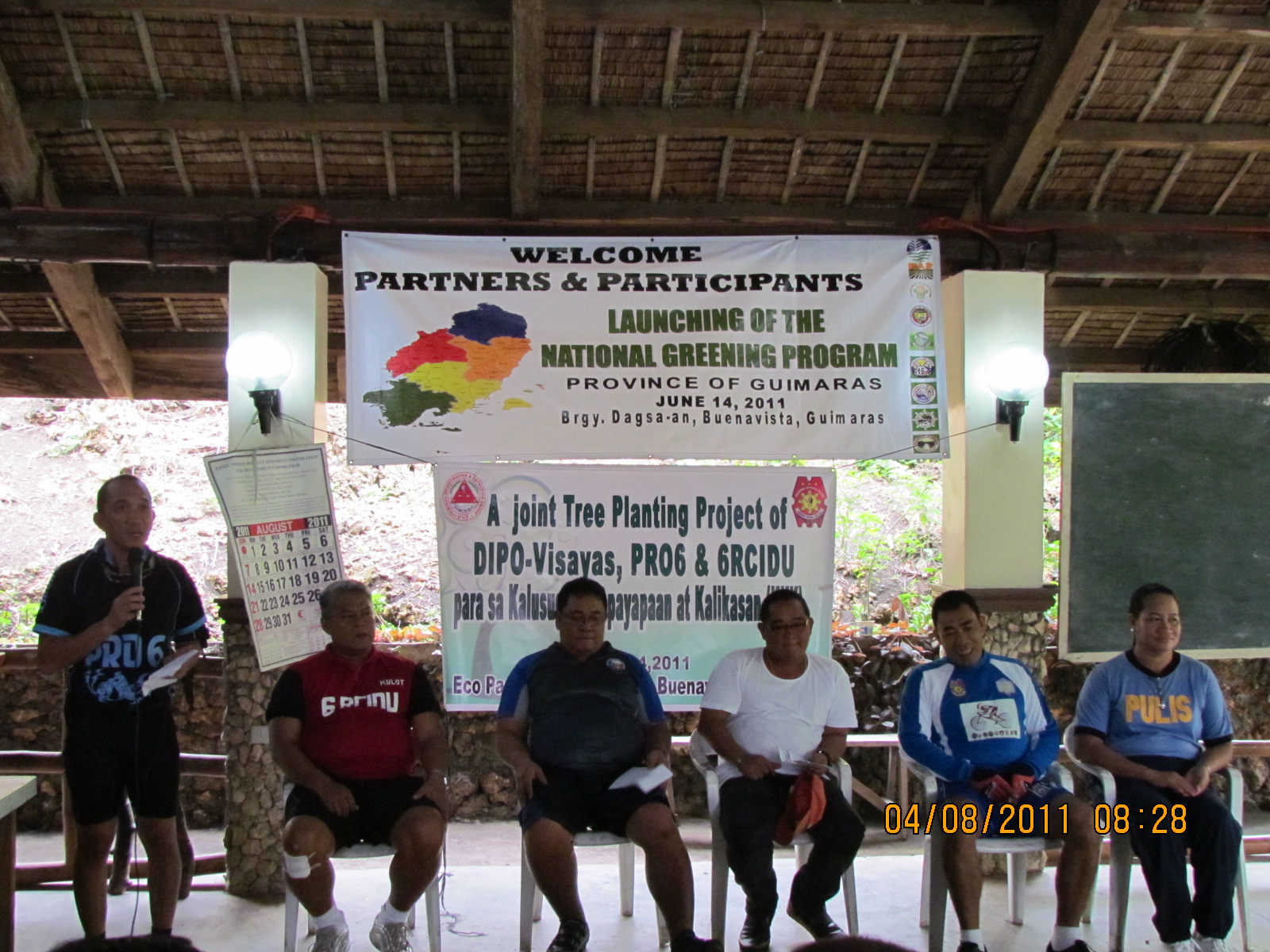The photograph captures an event, likely a ceremony or meeting, commemorating the launch of the National Greening Program. It features six men, five of whom are seated on white plastic patio chairs, while the sixth man stands on the far left, holding a microphone and a piece of paper, wearing a black shirt and black shorts. The event takes place in a roofed outdoor setting, characterized by white columns adorned with light bulbs, with an open wall that reveals greenery and a hill in the background. The roof overhead is wooden and brown.

Prominently displayed in the background are two white banners. The top banner reads: "Welcome partners and participants, launching of the National Greening Program, Province of Guimaras, June 14, 2011." The bottom banner describes the initiative as "a joint tree planting project of Depot Visayas and GRC IDU." The participants, dressed in casual clothing mainly consisting of T-shirts and shorts, appear to be addressing an unseen audience, suggesting an interaction or discussion about the program's objectives. Additionally, the backdrop features a blackboard and various signs, contributing to the setting's informative atmosphere.